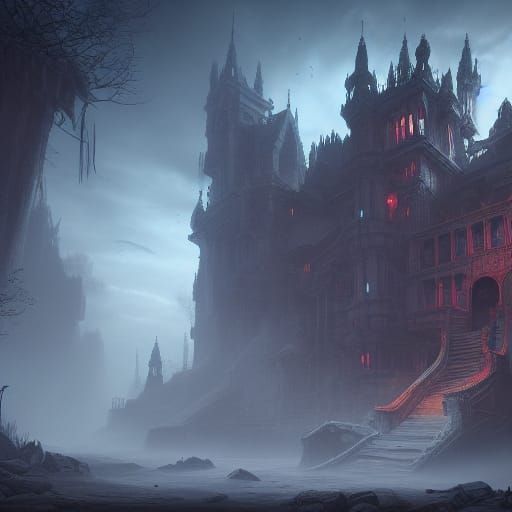The image is a digitally drawn, square depiction of a large and imposing medieval castle set against a stormy, overcast night sky filled with dark, swirling clouds. The setting is intensely spooky and gothic, further accentuated by fog that envelops the multi-storied structure. The castle itself stands several stories high, its numerous pointed towers adorned with long metal weather vanes. The right side of the castle is bathed in an eerie red light, while the left side fades into dark shadows. Red lights emanate from various windows and doorways throughout the castle, enhancing the foreboding atmosphere.

A long staircase, gray with touches of orange and dark red, leads up to an arched doorway, underlining the entrance's dramatic presence. The foreground features a rocky coastline with a crashed boat near the bottom right corner, adding to the scene’s sense of desolation. Dead, decaying trees frame the top left corner, silhouetted against the sky. The overall scene is shrouded in darkness and mystery, capturing a sense of fear and awe, reminiscent of gothic horror and medieval lore.